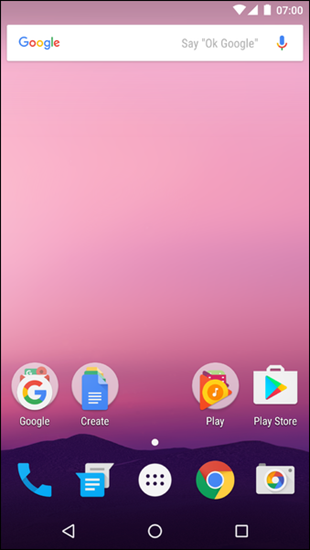This image is a high-resolution screenshot of a mobile phone's home screen, featuring a visually appealing gradient background transitioning from pink to purple. At the base of the image, there is a silhouette of dark purple mountains, lending a serene, artistic touch to the overall design.

At the top of the screen, a white rectangular Google search box prominently displays the text "OK Google" beside a microphone icon, indicating voice search functionality. Adjacent to this on the upper-right hand corner, three white filled-in icons display the device’s status information, including the time which is set at 07:00.

The main home screen is organized into a 3x3 grid of icons, beginning from the halfway point of the image. The first row includes four icons: 

1. **Google** - Represented by a multi-colored "G" within a white circle.
2. **Create** - Depicted with a blue text pad icon.
3. **Play** - Shown as a triangular-shaped orange button with a yellow circle.
4. **Play Store** - Displaying the characteristic Google Play ‘play’ button.

At the bottom center of the screen, five frequently used app icons are positioned:

1. **Telephone** - Depicted with a classic blue telephone receiver icon.
2. **Messages** - Represented by a white speech bubble icon.
3. **Navigation** - Shown as a blue arrowhead icon.
4. **Google Chrome** - Exhibiting the recognizable multi-colored circle.
5. **Google Photos** - Displayed with the multicolored pinwheel icon.

Further down, the image concludes with the device's navigation bar, which includes three essential buttons:

1. **Back** - A traditional triangle pointing left.
2. **Home** - A simple circle icon.
3. **Recent Apps** - Represented by a square icon.

The meticulously organized layout and cohesive color scheme offer a clean, user-friendly interface.